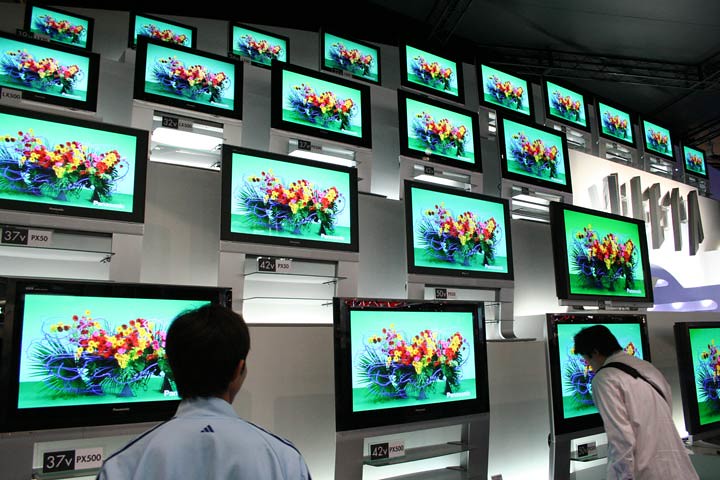This image shows an elaborate television display inside an electronics store, focusing on a variety of Panasonic Viera TVs. The TVs are arranged on a large wall in rows and columns, featuring screen sizes that range from 32 to 50 inches. Each screen displays a vibrant, colorful flower pattern that includes yellow, red, and pink flowers surrounded by green ferns and foliage, all set against a green backdrop. Below each television, there are tags indicating the model number and size, displayed in a combination of white text on black and black text on white.

In the foreground, there are two men examining the TVs. One man, wearing a blue Adidas tracksuit jacket with stripes on the sleeves, has longish dark hair and is bending over to get a closer look at one of the screens. The other man, standing upright, has a backpack or a bag slung over his shoulder and wears a white coat. The setup suggests an attempt to emphasize the technological prowess and visual capabilities of the Panasonic Viera TV models. Additionally, illuminated glass panes beneath the TVs and giant letters in the right corner of the display add a touch of sophistication and draw attention to the promotional setup.